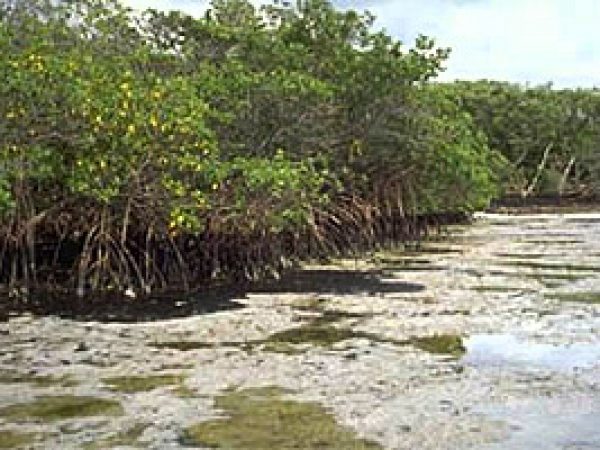This photograph, taken outdoors during the early daytime or noon, captures a bright and well-illuminated scene, albeit in low quality with some pixelation. In the upper right corner, a brilliant blue sky with a sprinkling of white clouds is visible. The upper half of the image is dominated by a dense canopy of green trees. The bottom half of the trees appears exposed, indicating that they were likely submerged underwater previously. These exposed roots create a stark contrast with the seemingly blackened area beneath, which may be either rotted wood or deep shadow—it is difficult to discern due to the image quality. In the lower portion of the photo, what seems to be a dried lakebed is marked by sporadic puddles of water, particularly noticeable in the right corner of the image.